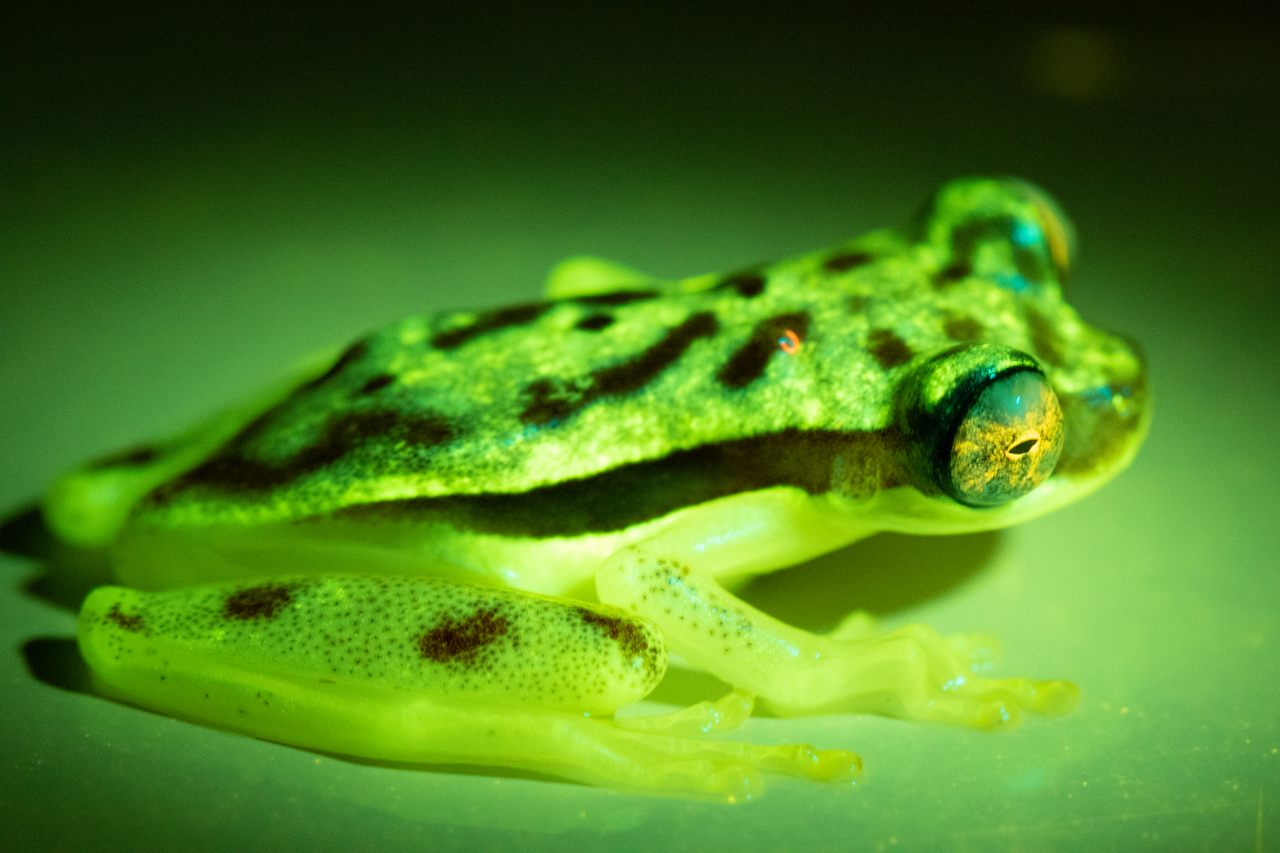The photograph captures a detailed, close-up image of a small green frog on a bright green surface, likely a leaf, though the lack of veins makes it indistinguishable. The frog, which appears to be a type of aquatic or tree frog found in tropical or jungle environments such as the Amazon, is light green with dark green and black markings. It is positioned facing to the right and slightly away from the camera, almost laying flat on its belly with one leg bent behind it. The frog's body features a prominent dark green stripe running from its nose, across its eye, and down its side, along with black spots on its back and legs. Its lighter-colored forelegs have black speckles. The frog's distinctive, bulging eyes are green with yellow streaks and small black pupils. Illuminated by a bright overhead light that casts a shadow underneath, the translucent, delicate parts of its anatomy, like its toes and arms, are subtly visible. The green background transitions from a lighter green at the bottom to a near-black dark green at the top, creating a contrast that emphasizes the frog's vibrant coloration.